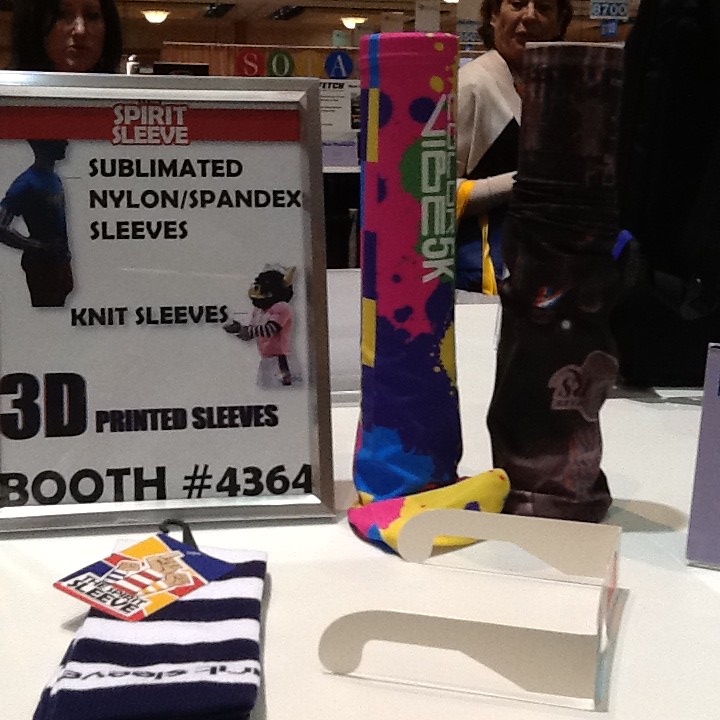In this detailed image, we observe a variety of objects meticulously arranged on a white table. Central to the display are several types of sleeves, prominently positioned in the middle of the image. These sleeves, identified as "spirit sleeves," come in different varieties including sublimated nylon spandex and knit sleeves, as noted on a propped-up sign. The sign also mentions booth number 4364 and shows images of a t-shirt and a stuffed animal.

Towards the bottom left of the table lies a sleeve with its tag still attached, while in the bottom right, we spot a pair of 3D glasses, likely paper versions. Upright, tube-like stands also hold additional sleeves. 

In the background, partly obscured, stand two people who appear to be in conversation or attending to the table. The whole scene is set indoors, suggesting a busy, possibly daytime event, potentially a flea market.

The array of colors featured includes white, black, dark blue, red, yellow, pink, purple, brown, and multiple shades that contribute to the vividness of the display. The collective details and the indoor setting suggest a lively, organized presentation of products.